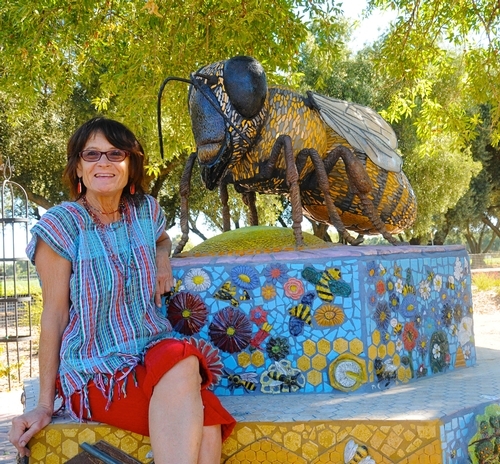The image shows a woman with brown hair sitting on a waist-high platform in an outdoor setting, possibly a park or playground, with children's play equipment visible on the left side. She is wearing red pants, a blue and red shirt, red earrings, and sunglasses, and she's smiling at the camera. Beside her is a large yellow and black bumblebee statue standing on a platform. The base of the platform includes a mural design with a blue background featuring hexagons, flowers, and smaller bumblebees. The scene is bathed in daylight with trees in the background catching most of the sunlight, and the sky appears to be a blend of white and green hues.